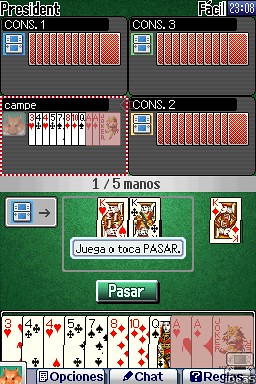This image is a screenshot from a digital card game. The game interface displays multiple shuffled decks arranged neatly along the bottom of the screen. At the top of the screen, there are three visible player avatars or icons, each likely representing an active player in the game. Situated around these avatars are more cards, positioned face down, ready to be played or drawn. In the top-left corner of the screen, the word "Precedence" is prominently displayed, suggesting a rule or turn order indicator within the game. The upper-right corner of the screen shows the current time, 23:08 (or 11:08 p.m.), indicating a late-night gaming session.